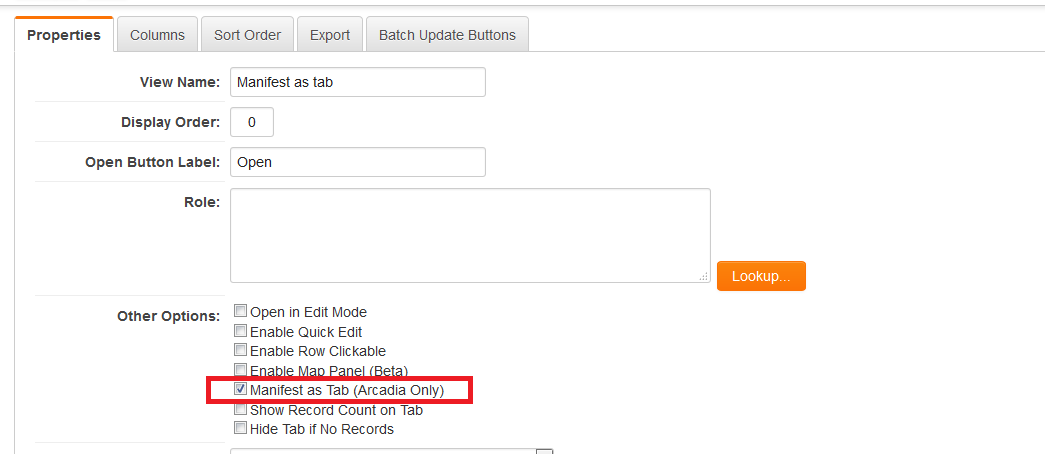A detailed screenshot of a computer screen displaying a multi-tab interface is shown. The interface features five tabs, with the first tab titled "Properties" highlighted by an orange line at the top and a white background. The remaining tabs—"Columns," "Sort Order," "Export," and "Batch Update Buttons"—have gray backgrounds without any highlighting.

Beneath these tabs, the text "View Name" is displayed adjacent to a text box containing the entry "Manifest As tab." Below this, the label "Display Order" is visible, accompanied by a text box with the numeral "0." Following this, there's the label "Open Button Label," with a text box containing the word "Open." Next, there’s a section titled "Rule," featuring a large, empty text box, followed by an orange rectangle button labeled "Look Up."

The section "Other Options" displays seven listed options, each accompanied by a checkbox. The checkboxes are predominantly empty except for one. The listed options and their respective checkbox statuses are as follows:

1. "Open in Edit Mode" - the checkbox is unchecked.
2. "Enable Quick Edit" - the checkbox is unchecked.
3. "Enable Rule Clickable" - the checkbox is unchecked.
4. "Enable Map Panel Beta" - the checkbox is unchecked.
5. "Manifest As Tab Arcadia Only" - the checkbox is checked and encased within a red border.
6. "Show Record Count on Tab" - the checkbox is unchecked.
7. "Hide Tab with No Records" - the checkbox is unchecked.

Each element on the screen is meticulously organized and clearly labeled, making the interface user-friendly and navigable.